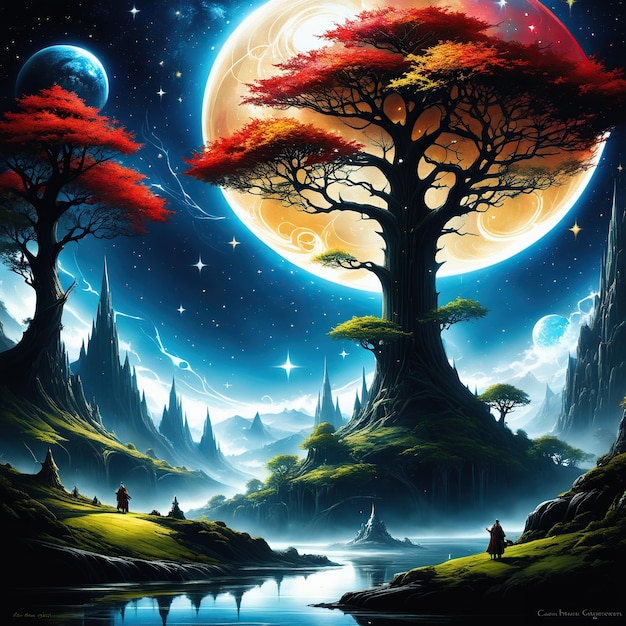This digital illustration, likely AI-generated, vividly depicts a fantastical, otherworldly landscape. Dominating the scene is a massive tree with a black trunk, rooted on an island in the middle of a water body. Its striking foliage, a mix of bright red and yellow leaves, is the central focus. The backdrop features a dark blue sky adorned with glimmering stars, some brighter than others, and an enormous, slightly distorted orange moon whose appearance suggests AI involvement. Another blue planet hovers in the upper left, enhancing the surreal atmosphere.

Surrounding the primary tree are smaller trees bearing similar red crowns. jagged, sharp-pointed rocks jut out of the vivid green grass that lines the water’s edge, adding to the otherworldly terrain. Two figures, possibly cloaked silhouettes, stand in awe on opposite sides of the water, each on a green hill. Further adding to the dramatic scenery are distant, grey, and sharp-peaked mountains piercing through clouds into the star-studded sky. A barely readable signature adorns the bottom of this image, emphasizing its unique, almost ethereal quality.